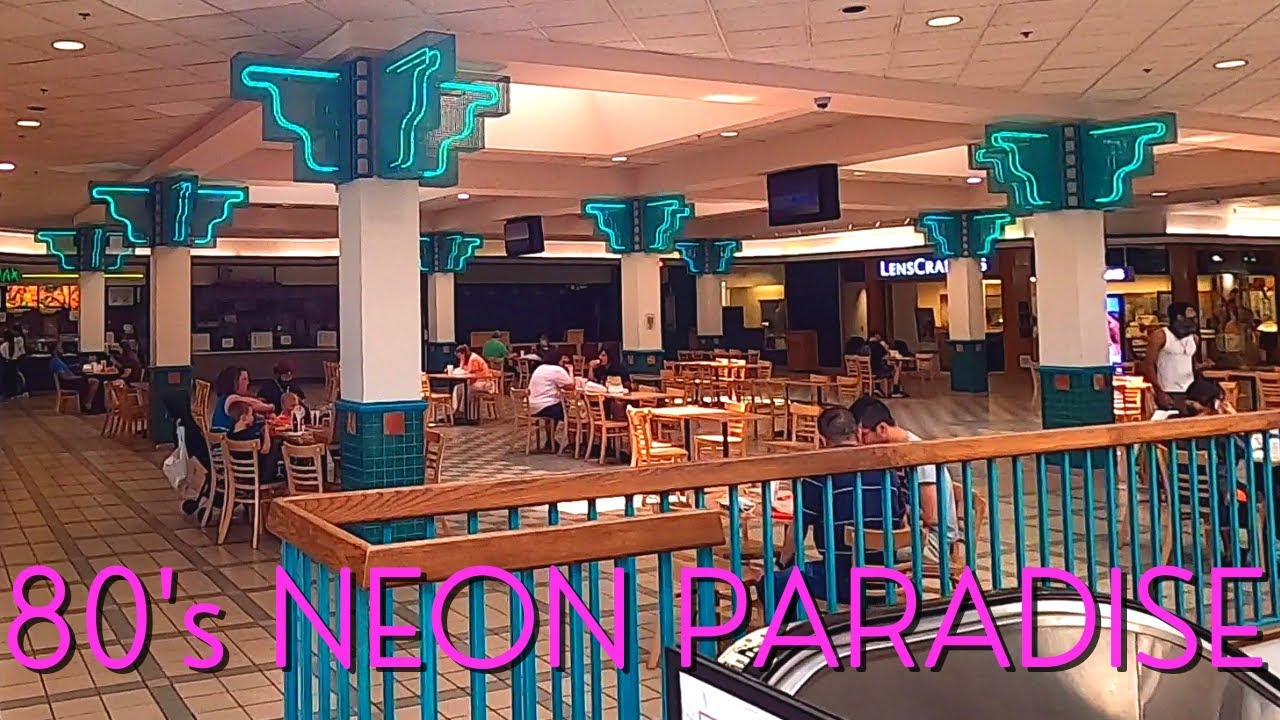The photograph depicts a vibrant food court in a mall, aptly named "80s Neon Paradise," as indicated by the bright, neon pink text at the bottom of the image. The scene is set on an old-fashioned tiled floor with tan and light brown stripes, lending a retro atmosphere. Prominent throughout the space are large square pillars, each about 18 inches wide, adorned with a teal green checkered design up to about three to four feet high and transitioning to white up to the ceiling. These pillars feature unique, upside-down staircase-like Tetris pieces, which are enhanced with neon lights, adding to the nostalgic decor.

The food court is spacious and filled with numerous wooden tables and chairs, varying from oak-colored to darker shades. An escalator is visible in the foreground to the right, with a teal and brown railing guiding visitors. Scattered around the tables, several groups of two to three people are seated, enjoying their meals. In the background, most of the storefronts are closed and dimly lit, except for one store partially visible beyond a pillar, named "Len's Crap." The overall ambiance reflects a lively yet nostalgic dining area, reminiscent of the 1980s.